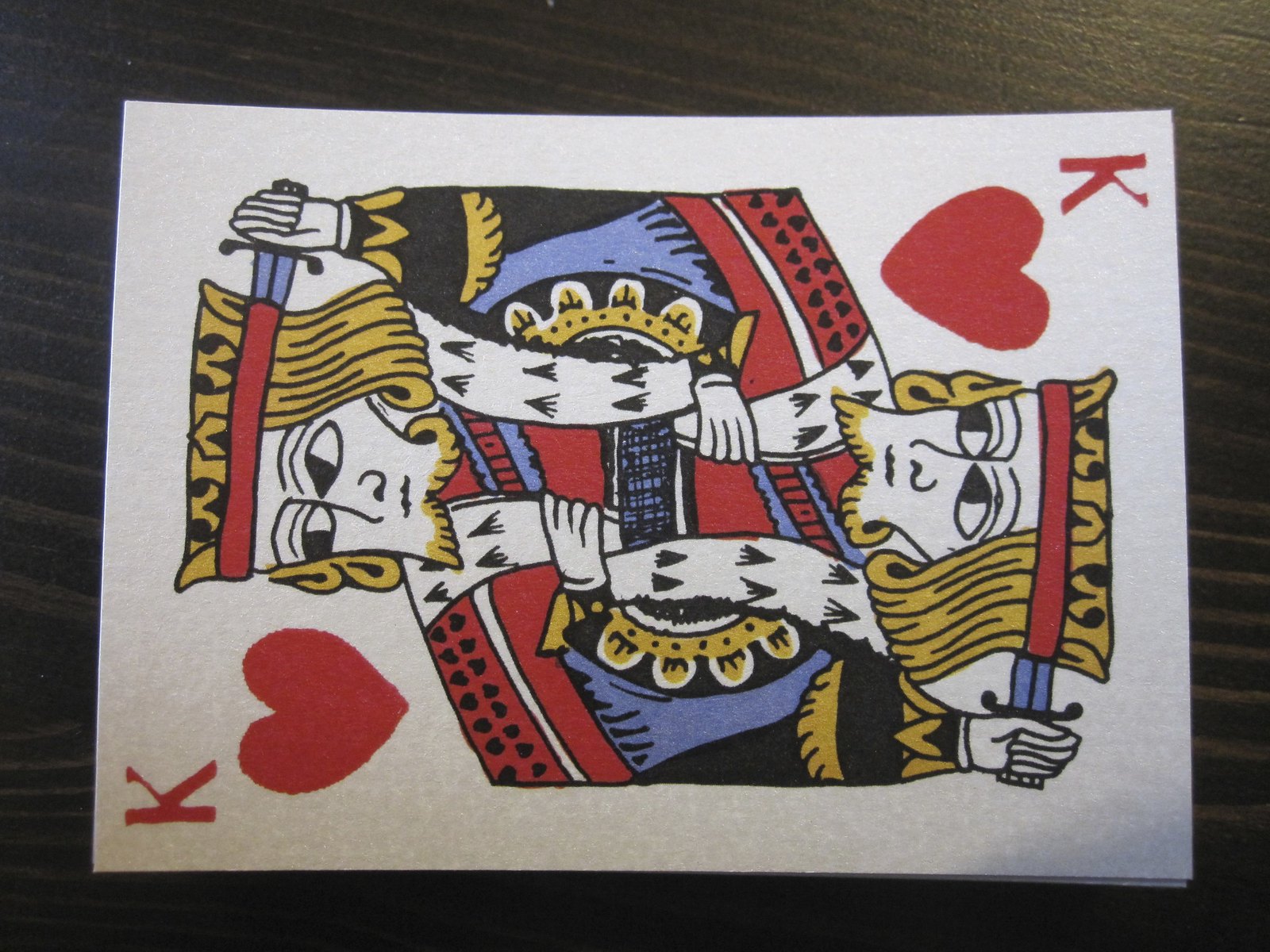The image showcases a close-up of an intricately detailed playing card, specifically the King of Hearts. The card appears almost like a painting due to its impressive size, though it might simply be a highly zoomed-in view, as evidenced by the visible wood grain of the brown table upon which it rests. The card is laid horizontally, with the "K" symbol in the bottom right corner and one of the king's heads oriented to the left. Conversely, another head faces rightwards with the corresponding "K" in the top right corner. The white canvas of the card features two regal kings adorned in red with yellow hair, each grasping a sword behind their heads and donning a white fur-lined coat. The design includes black and white type motifs, adding an elegant touch. Notably, the hearts on the card exhibit an almost bleeding effect, with their edges appearing jagged and uneven. Additionally, a subtle white spot is visible at the bottom part of the left king figure, revealing part of the surface beneath the card.